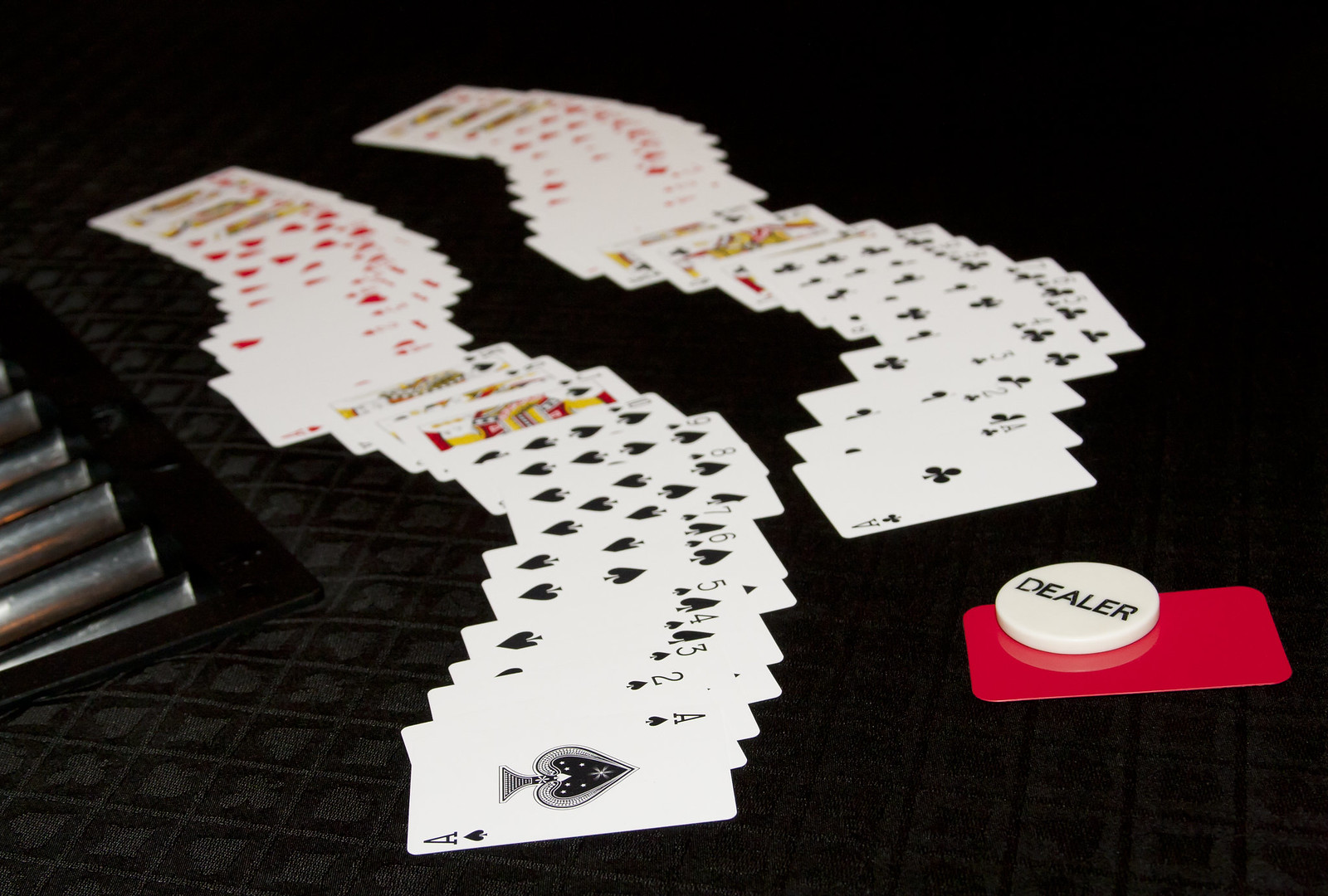This image depicts a busy betting station filled with various gaming elements. At the bottom right, a solid red, rectangular card is positioned diagonally. On this card, a circular object prominently displaying the word "DEALER" in black text on a white background can be seen. To the far left, a metallic structure with several horizontal, silver-colored cylinders is present, likely used for holding coins. Below this structure, in the bottom middle left of the image, is a table with a black surface adorned with numerous small logos in the form of spades, hearts, and diamonds, all in a light grayish color.

In the center of the image, a spread of playing cards is arranged horizontally, though the perspective is slightly skewed to the right, giving them a diagonal orientation. The cards are laid out systematically, showing a full sequence from Ace to King for both black and red suits. The bottom middle section displays the black suits vertically, while the red suits are arranged horizontally beside them. The same pattern is repeated above with the clubs. The overall scene captures the essential components and atmosphere of a betting station, emphasizing the organized array of cards and the functional elements used in the betting process.